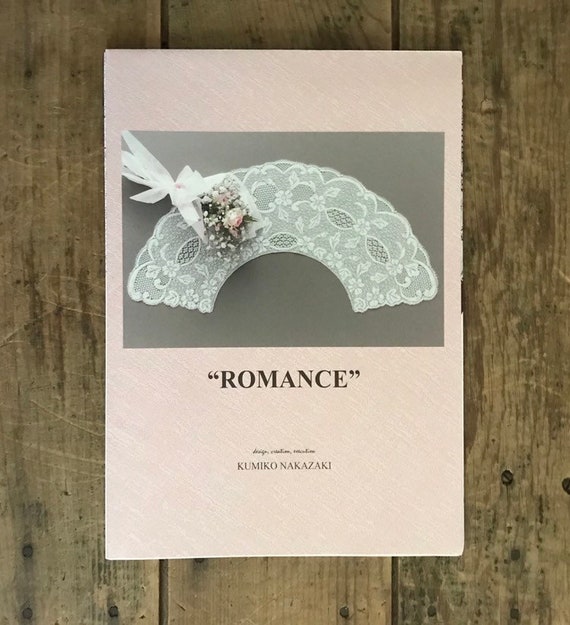The photograph features a background of brown wooden panels with three vertical lines running through them, secured with visible nails. Mounted on this wall is a very light pink sheet of paper. At the center of this paper is a dark gray rectangular box. Within this gray rectangle, there is a photo showcasing a white lace semi-circle adorned with a flower arrangement of pink roses. Below this decorative lace image, the word "ROMANCE" is prominently displayed in bold, all-caps black font. Accompanying this, smaller text reads "Kimiko Nakazaki" followed by the words "design, creation," and possibly "installation," though the font size makes it difficult to confirm the final word. The overall presentation appears to emphasize romantic aesthetics.